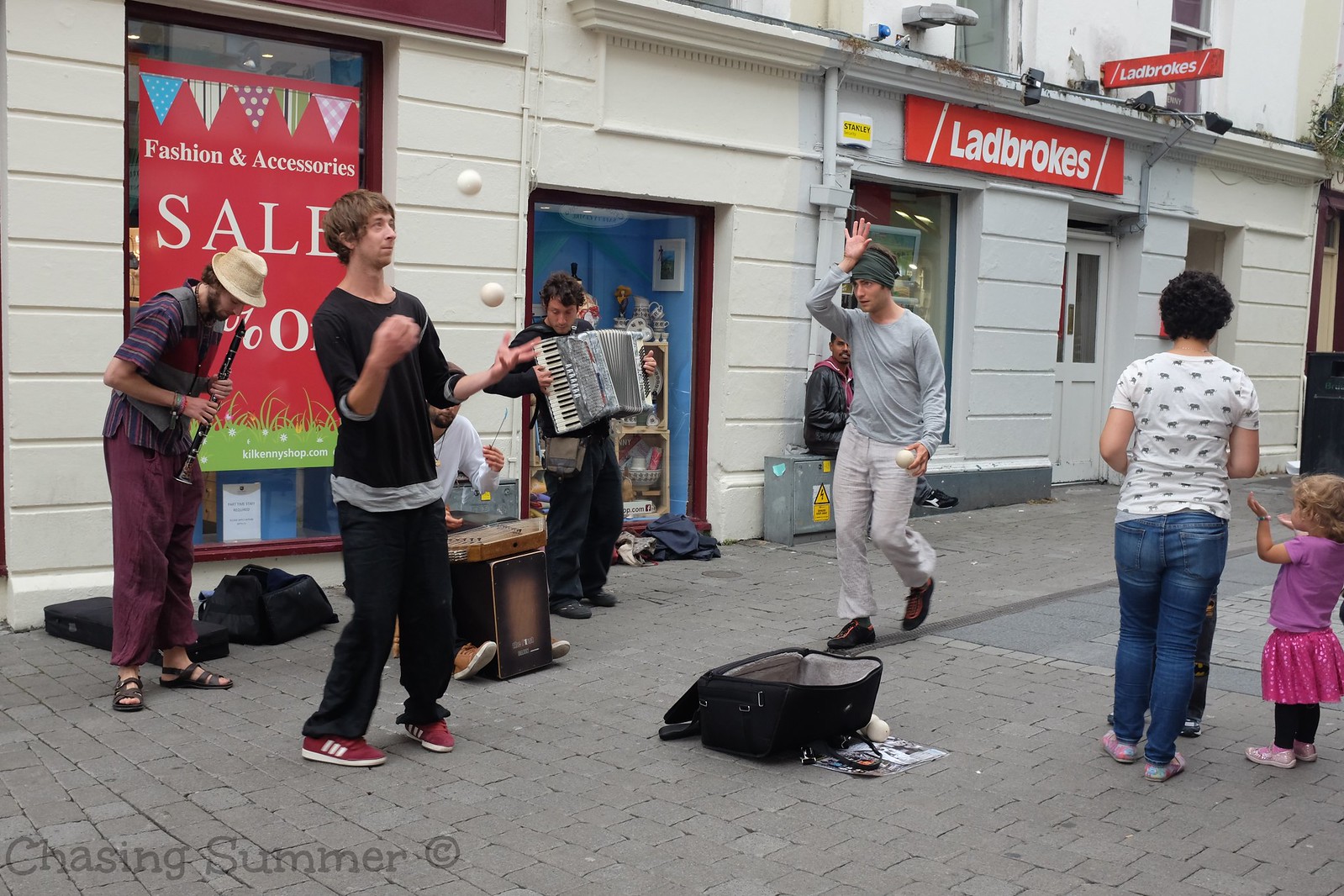The color photograph titled "Chasing Summer ©" captures an animated street scene on a gray brick sidewalk in front of a white brick building. In the foreground, several buskers are performing, infusing life into the scene. On the far left, a man dons sandals, purple pants, and a striped collared shirt under a vest, topped with a white hat, as he skillfully plays a clarinet. Beside him, a man in black with red sneakers energetically dances. Another musician, also dressed in all black, plays an accordion. 

The backdrop features a brightly colored storefront with a prominent red sign advertising a "Fashion and Accessory Sale," embellished with small triangular banners in various patterns, including blue, striped, and polka dots, above green grass and small flowers in white and yellow. Above this sign, the store name "Ladbrokes" is displayed in large white letters bookended by two slashes.

As part of the lively backdrop, a passerby—dressed in a gray shirt, white pants, and dark shoes—walks by with his hand on his head. In the scene, there is also an open suitcase on the sidewalk and a woman with a small child in tow. The woman is in a white shirt and blue jeans, while the child wears a purple shirt, pink skirt, and black leggings. Another observer, clad in a black leather jacket and purple shirt, sits nearby on what appears to be an electrical box. The composition masterfully captures the dynamic essence of street performance against the vibrant urban setting.